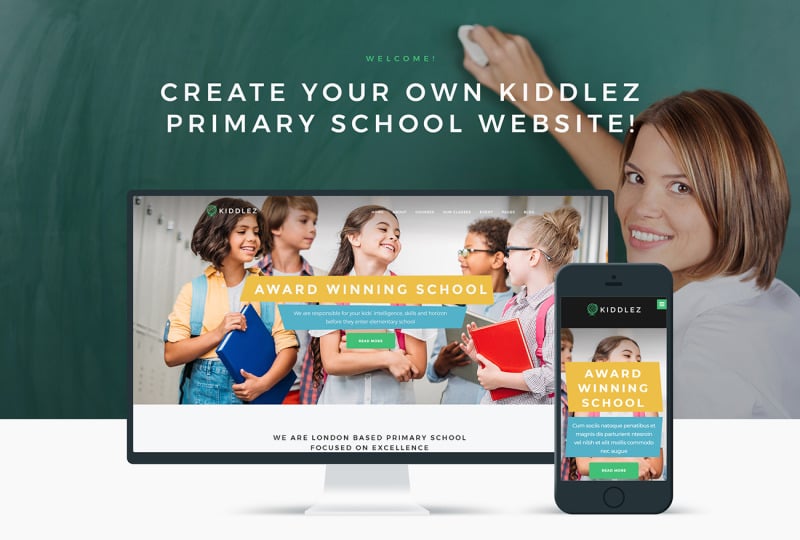The image displays a website with a chalkboard-themed background, characteristic of a traditional green board that has been erased multiple times, creating white streaks. Positioned to the right is a woman with her right arm raised, holding chalk against the board. Above, "WELCOME" appears in small, green, uppercase letters. Below, larger white text reads, "Create your own Kiddus Primary School website," with the word "Kiddus" possibly spelled "K-I-D-D-L-E-S" or "K-I-D-D-L-E-Z."

Central to the image is a graphic of a computer monitor with a black trim and a silver base. Displayed on the screen are five children smiling, situated within a school setting. Over them is a gold banner with the inscription "Award-Winning School" in white text. Directly beneath this is a blue banner, accompanied by a green button labeled "Sign Up."

At the bottom of the image, a white text states, "We are a London-based primary school, focused on excellence." Adjacent to the monitor, a cell phone screen features a close-up of one of the children's faces, overlaid with the same gold and blue banners and green "Sign Up" button, consistent with the design elements on the website.